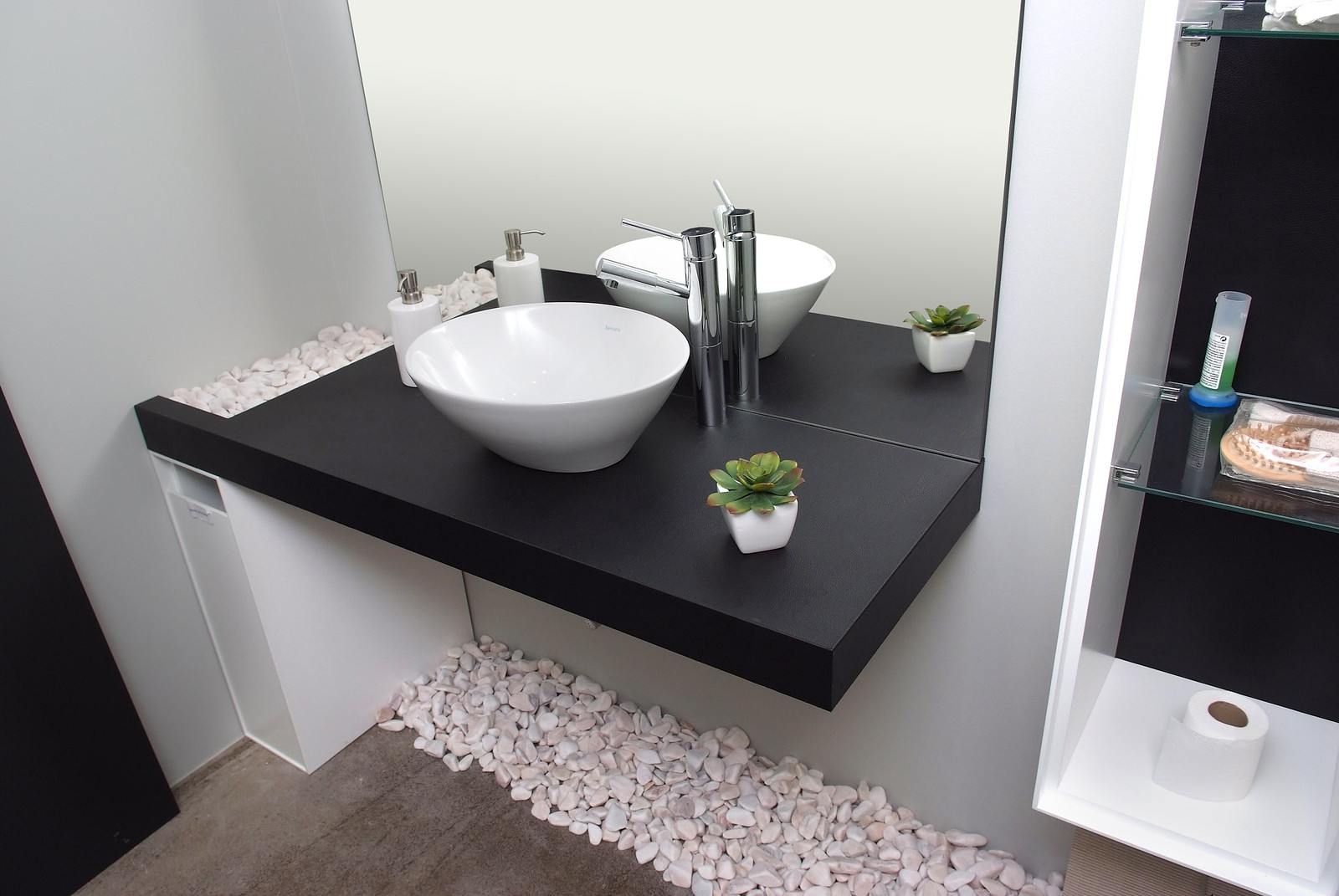The image depicts a high-end, modern bathroom characterized by an unusual and striking design. The walls are gleaming white or pale gray, illuminated by a crisp, diffuse white light that enhances the room's sleek aesthetic. The floor has a weathered gray appearance, reminiscent of wood often found in beachside towns, although it's unclear if the material is tile, vinyl, or concrete.

A black countertop with a floating design extends from the wall, supported on the left side by a narrow, white, and sleek cabinet. Beneath the counter, a small section of plumbing is visible. Atop the counter rests a round white porcelain vessel sink, complemented by a tall, sleek chrome faucet. One notable feature is the left edge of the counter, which ends in a trough filled with white pebbles, adding a unique, decorative touch.

Beneath the sink, between the gray floor and the wall, lies another row of pebbles, resembling an indoor garden bed. These pebbles are not grouted but appear to be loosely poured into place, creating an unexpected indoor-outdoor blend.

A wall-mounted mirror hangs above the sink, while a small potted succulent in a square white ceramic pot adds a touch of greenery to the minimalist space. On the right side of the photo, an open shelving unit floats against the wall, framed in white with a black-painted back and glass shelves. Toilet paper is visible on the bottom shelf, though the contents of the other shelves remain unidentified.

The combined elements of sleek surfaces, unexpected natural features, and modern fixtures create a distinctive and luxurious bathroom setting.